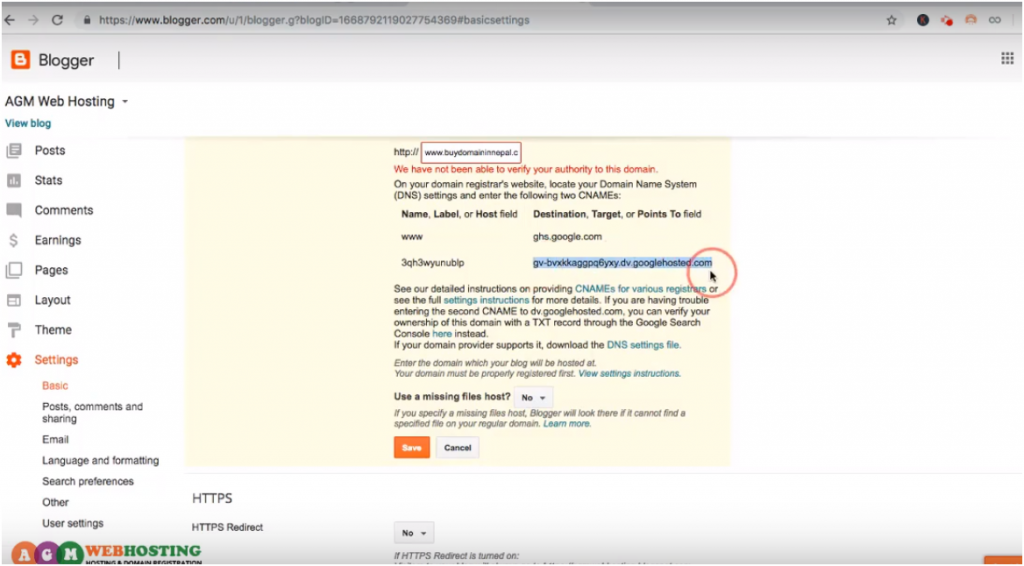This image showcases a Blogger website interface. In the top left corner, the distinctive Blogger logo is prominently displayed; it features an orange square with a white 'B' in the center. On the left side of the interface, there is a vertical menu offering various navigation options: Posts, Stats, Comments, Earnings, Pages, Layout, Theme, and Settings. Within the Settings menu, additional options are listed in black text, including Posts, Comments, Sharing, Email, Language and Formatting, Search Preferences, and Other User Settings.

The main content area of the webpage currently displayed has a yellow background, contrasting with other sections of the interface, which have a white background. At the top of this page, there's an HTTP URL box. Below the URL box, a red text notification reads, "We have not been able to verify your authority to this domain." Following this notification is a section of text providing further information or instructions. At the bottom of this section are two buttons: a Cancel button and a Save button, the latter of which is orange with the word "Save" written in white.